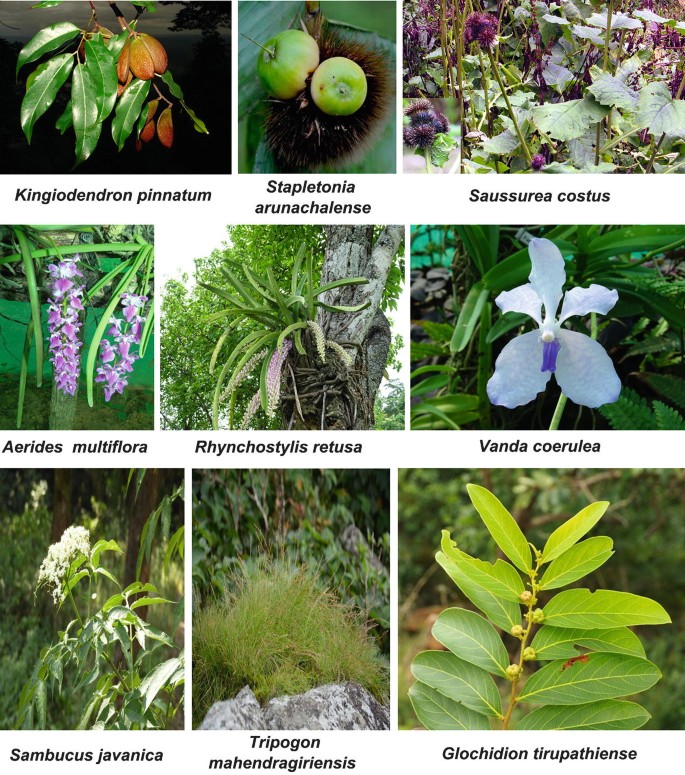This vertical rectangular image serves as an informative chart, showcasing various wildflowers along with their Latin names. Arranged in three rows, each row contains three images, resulting in a structured and visually appealing format. The floral images include different flowers and leaves, making it both educational and aesthetically pleasing. 

Starting from the top left corner, the first image depicts Kingiodendron pinnatum; it features some leaves and a fruit-like hanging flower with thick brown petals. Next to it, in a square format, is the Stapletonia aurunchalens, which appears as two apple-like structures on a spiny bush attached to a large leaf. The third image in the top row, a rectangle on the right, presents Zassaria costus with distinctive black spiny balls in clusters atop a thick green stem.

In the second row, the first rectangular image highlights various bell-shaped flowers, though their exact species name isn't specified in the original descriptions. Details on the rest of the flowers in this row are sparse in the provided voice notes.

Finally, the lower row includes a notable example: Glowchydian pyrrhopsymensa. This plant features green leaves flanking a central stem adorned with small, berry-like structures. 

The chart is filled with Latin names, making identification challenging for those without botanical expertise, but it offers a rich visual reference for enthusiasts and learners alike.